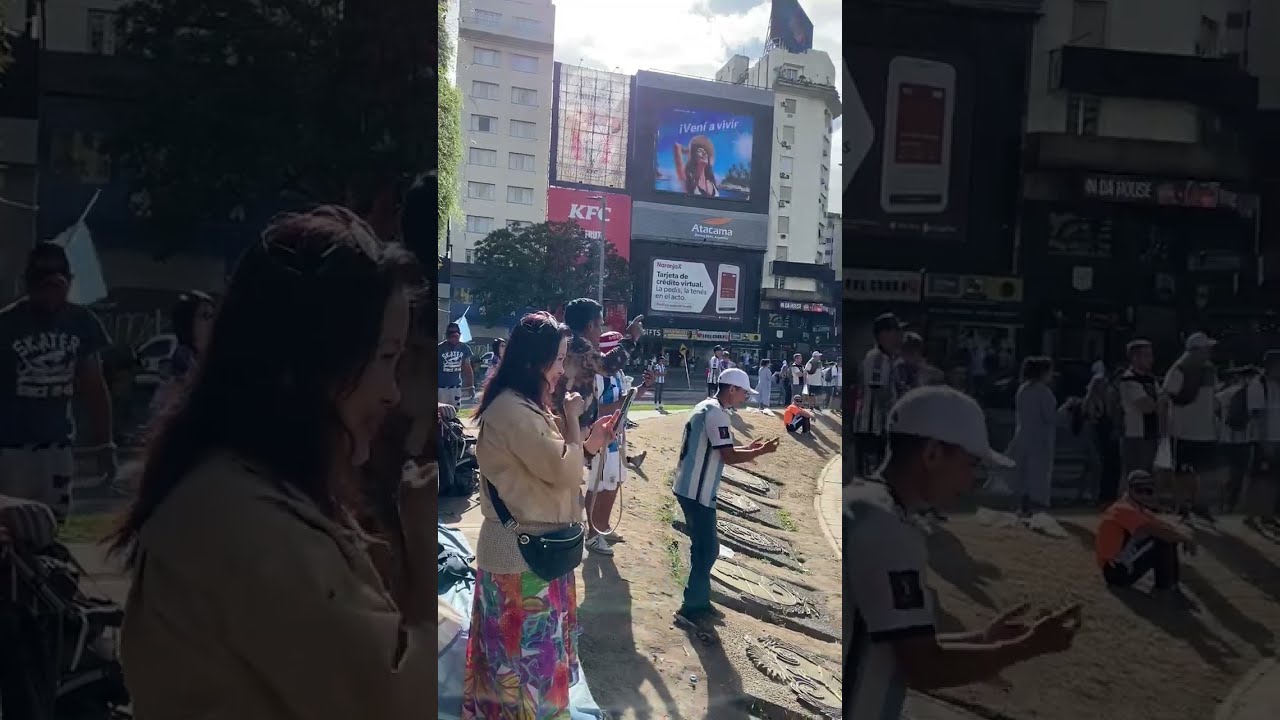The image captures an outdoor scene in a bustling cityscape. In the foreground, four people are gathered on a sandy hill, with two prominently facing to the right. One woman, wearing a colorful skirt and a brown top with a bag draped across her, stands out with her long, dark hair. Nearby, a man in a blue and white striped shirt, a white cap, and blue jeans is visible. The sun casts clear shadows, indicating a sunny day. To the right of this group are several concrete plaques with images on them. In the background, a street populated with more people extends into the distance, bordered by multi-story commercial buildings adorned with advertisements. One prominent sign is for KFC, while another building boasts a large electronic billboard displaying an ad. Above the scene, a tree spreads its branches, adding a touch of greenery. The sky is partially visible, dotted with white clouds. The image has a distinctive border created by enlarging and graying out elements from the central image.